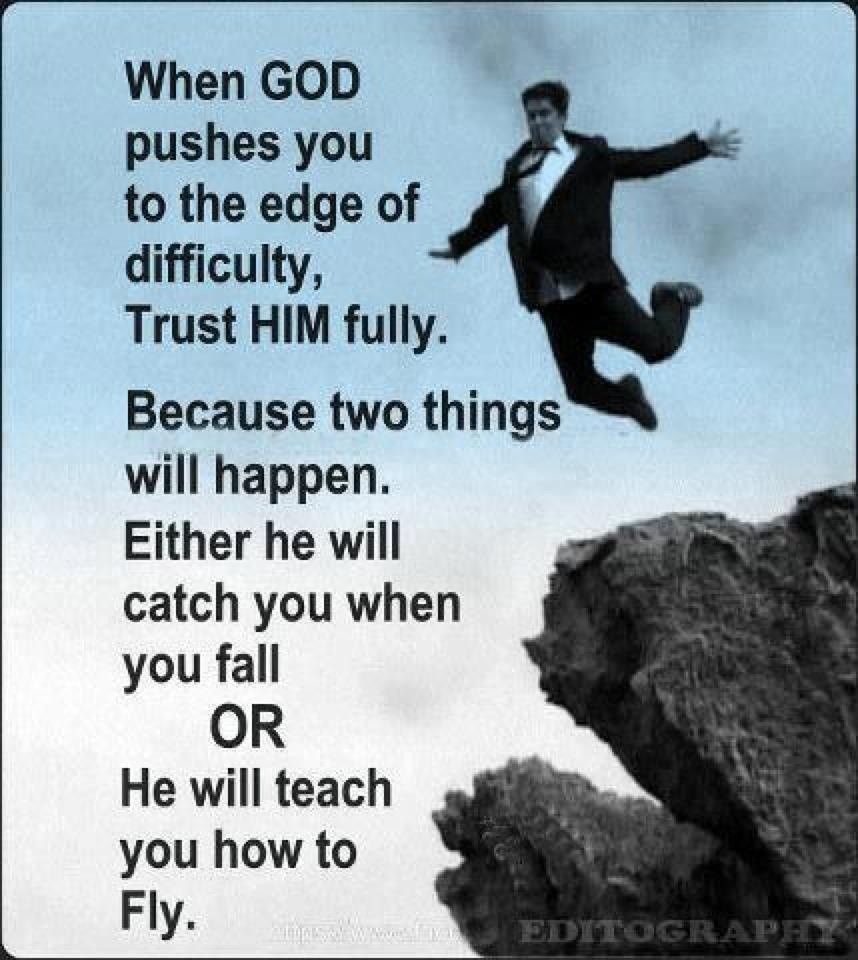The image portrays a monochromatic, motivational poster, tinted in blue and white hues, emphasizing a religious message. Set against a gradiated sky, transitioning from white at the bottom to blue at the top, a man in a suit and tie leaps off a cliff, emanating a sense of trepidation visible in his concern-filled expression. His arms are extended outwards, chest puffed, with his legs stretched behind him and his tie flapping in the air. To the left of the image, in bold black text, is an inspirational quote: "When God pushes you to the edge of difficulty, trust Him fully. Because two things will happen. Either He will catch you when you fall, OR He will teach you how to fly." In the bottom right corner, transparent text reads "editography," and the entire image is framed with a subtle black border. The rocky cliff emerges from the bottom right, grounding the dramatic leap amidst an expansive sky.